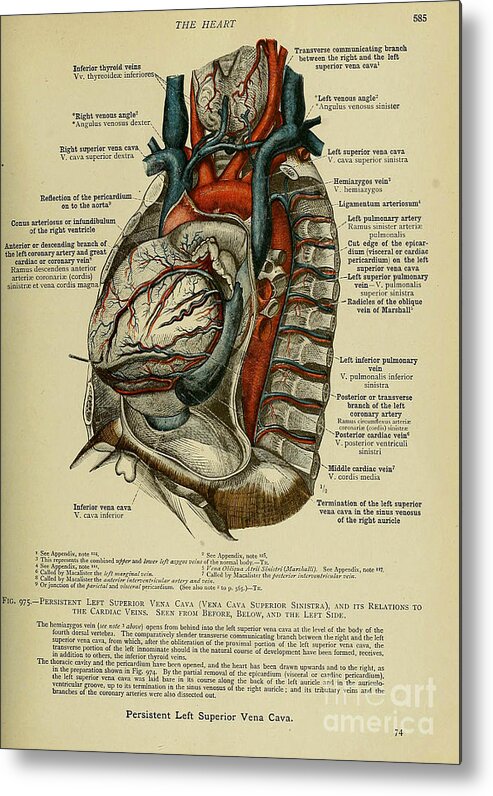The image is a detailed, colorful scientific illustration of a human heart, depicted in a lateral view exposing various anatomical features alongside the ribs. The background is a pale beige, which accentuates the intricate details and labeling. The heart illustration utilizes a color scheme with red and blue to indicate different blood flows, while other parts are shown in grayscale. The top of the image bears a small-font title, "The Heart," alongside a page number, "585," in the top right corner. Extensive labeling of the heart's structure includes terms like the anterior thyroid veins, right superior vena cava, left superior vena cava, and persistent left superior vena cava, among others. Additional paragraphs of small-font explanatory text are positioned below the diagram. At the bottom of the page, the text "Persistent Left Superior Vena Cava" is clearly labeled, with the number "24" on the bottom right, and the Fine Art America watermark in the lower right corner.